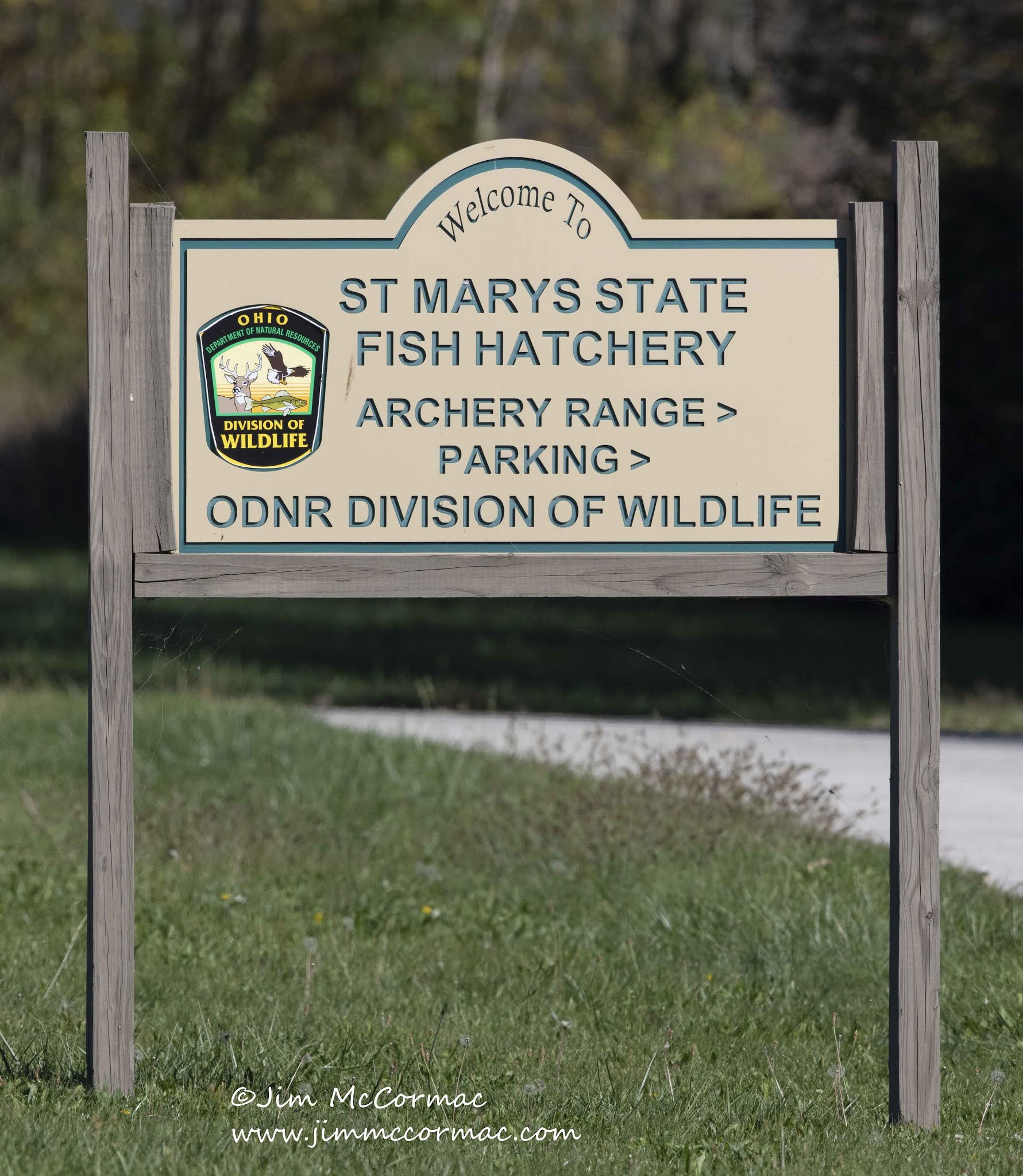A photograph taken by artist Jim McCormick, identifiable by his watermark and website at the bottom of the image, showcases a vibrant scene of nature interspersed with details that captivate the viewer. In the foreground, an array of grasses dominates the scene, ranging from light to dark green, punctuated by a sparse sprinkling of tiny yellow flowers situated near the center.

The focus of the image is a prominent sign, mounted on a wooden post of weathered gray tones. The sign itself is constructed from tan-colored wood and is framed by a bluish border that complements the blue font of the text. Adding to its rustic yet official look, the sign features a detailed medallion to one side in shades of gold and green. This emblem depicts an antlered animal alongside a soaring bird, encapsulated by the word "Ohio" in gold and additional green text below. At the base of the medallion reads "Division of Wildlife" in yellow.

The main text on the sign warmly welcomes visitors to "St. Mary's State Fish Hatchery" and provides directions for "Archery Range Parking," along with acknowledging its administration by the "ODNR Division of Wildlife." This carefully composed image not only conveys detailed information but also enriches the essence of the natural setting.